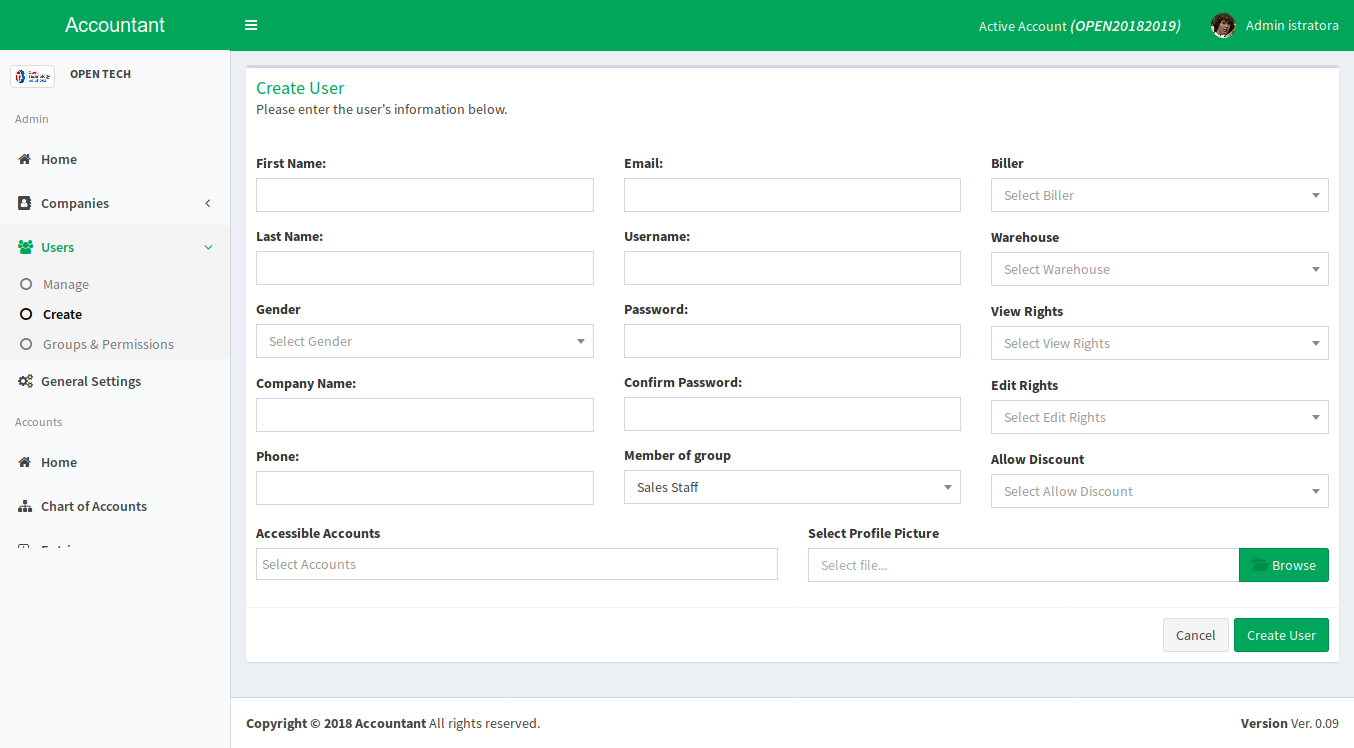The image is a screenshot of a web page dedicated to user creation within an accounting software interface. At the very top of the page, there is a thin green bar. On the top left-hand side, the word "Accountant" is displayed in white text. On the top right, it reads "Active Account (Open 2018-2019)" alongside the name "Administrator" and a profile picture of a woman with curly brown hair.

The left-hand side of the screen features a vertical gray navigation column. At the top of this column, "Open Tech" is written, followed by various categories listed below: Home, Companies, Users, Manage, Create, Groups and Permissions, General Settings, Accounts, Home, and Chart of Accounts.

On the right side, the background is grayish with a white rectangle embedded within. The top left corner of this white rectangle contains green text reading "Create User," accompanied by the instruction, "Please enter the user's information below." Beneath this, various input fields are arranged left to right, top to bottom: First Name, Email, Biller, Last Name, Username, Warehouse, Gender, Password, View Rights, Company Name, Confirm Password, Edit Rights, Phone, Member of Group, Allow Discount, Accessible Accounts, and Select Profile Picture. A green "Browse" button accompanies the profile picture field. 

At the bottom of the page, there are two actionable buttons – "Cancel" on the left in gray and "Create User" on the right in green.